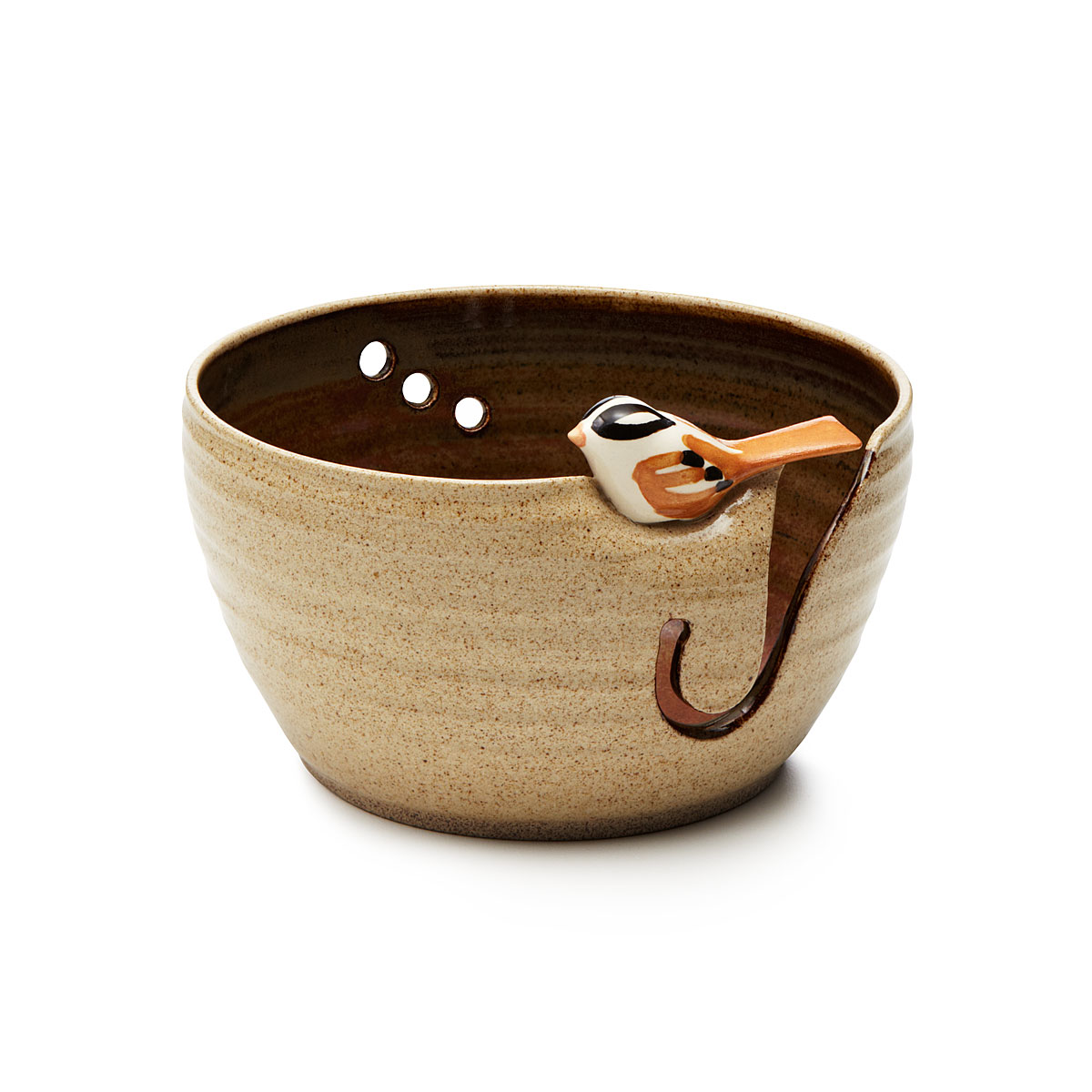In this photograph, there is a ceramic cup or small mug set against a completely white background. The ceramic piece has a light beige, tan, or sandy-colored exterior adorned with darker brown speckles and vertical striations, providing a textured appearance. Prominently, a small ceramic bird with a white body, black eye markings, and light brown feathers, beak, and tail is perched on the rim of the mug. The interior of the mug is a contrasting dark brown and features three horizontal holes on the far side. Interestingly, the mug has a distinctive design with a curvy, J-shaped section or "curly Q" on the right side, making it unsuitable for holding liquids. This unique combination of elements, including the bird and the unusual carved section, creates an intriguing and eye-catching ceramic artwork.